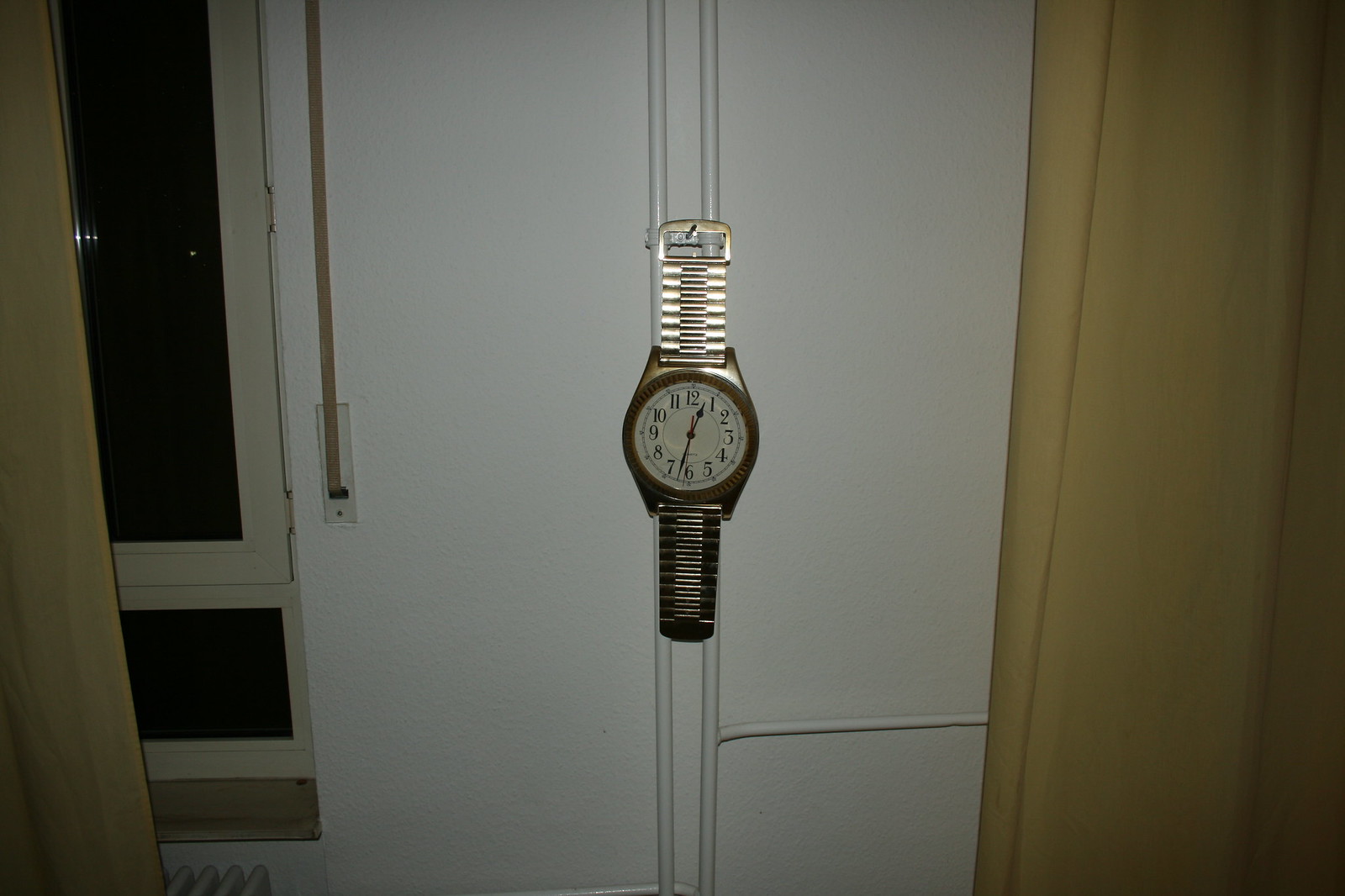This photograph captures a dimly lit room, where a gold watch hangs prominently from a small nail on a white wall. The center of the image is dominated by two thin, white-painted poles that extend vertically out of the frame. The gold watch, suspended towards the upper-central part of the image, features a white face with black numerals indicating the time as 12:32. On the right side of the photograph, a yellow curtain partially covers the scene, spilling over to the left where it is pulled back to reveal a window behind it. The stark contrast between the bright gold watch and the muted tones of the room enhances the watch’s prominence, creating a focal point amidst the obscured shadows.